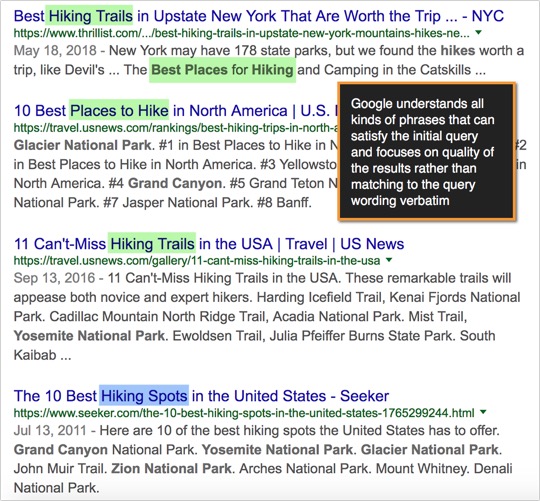The image features a stark white background, intricately detailed with blue lines that structure the layout, while the text is presented in black. At the center, there is a prominent black box with an eye-catching gold outline, containing white print. The text within the box reads: "Google understands all kinds of phrases that can satisfy the initial query and focuses on quality of the results rather than matching the query wording verbatim."

At the top, highlighted in blue, is the phrase "best hiking trails," which is followed by the description "in upstate New York that are worth the trip," and it includes the source website in green. Another section reads, "New York may have 178 parks but the best places for hiking," with the phrase "hiking trails" enclosed in a green box. 

Further down, a blue-highlighted title states "10 best places to hike" within a green box, listing notable locations such as Glacier National Park, Grand Canyon, and Yellowstone. Next, the caption includes "can't miss hiking trails," with the term "hiking trails" highlighted in green, attributing the information to Travel US News.

Lastly, there is a segment labeled "10 best hiking spots," boxed in blue, within the United States. This segment is sourced from Seeker and highlights famous spots like the Grand Canyon and Zion National Park, among others. 

This visually engaging image comprehensively showcases Google’s ability to provide quality search results that go beyond a mere verbatim match to the query.